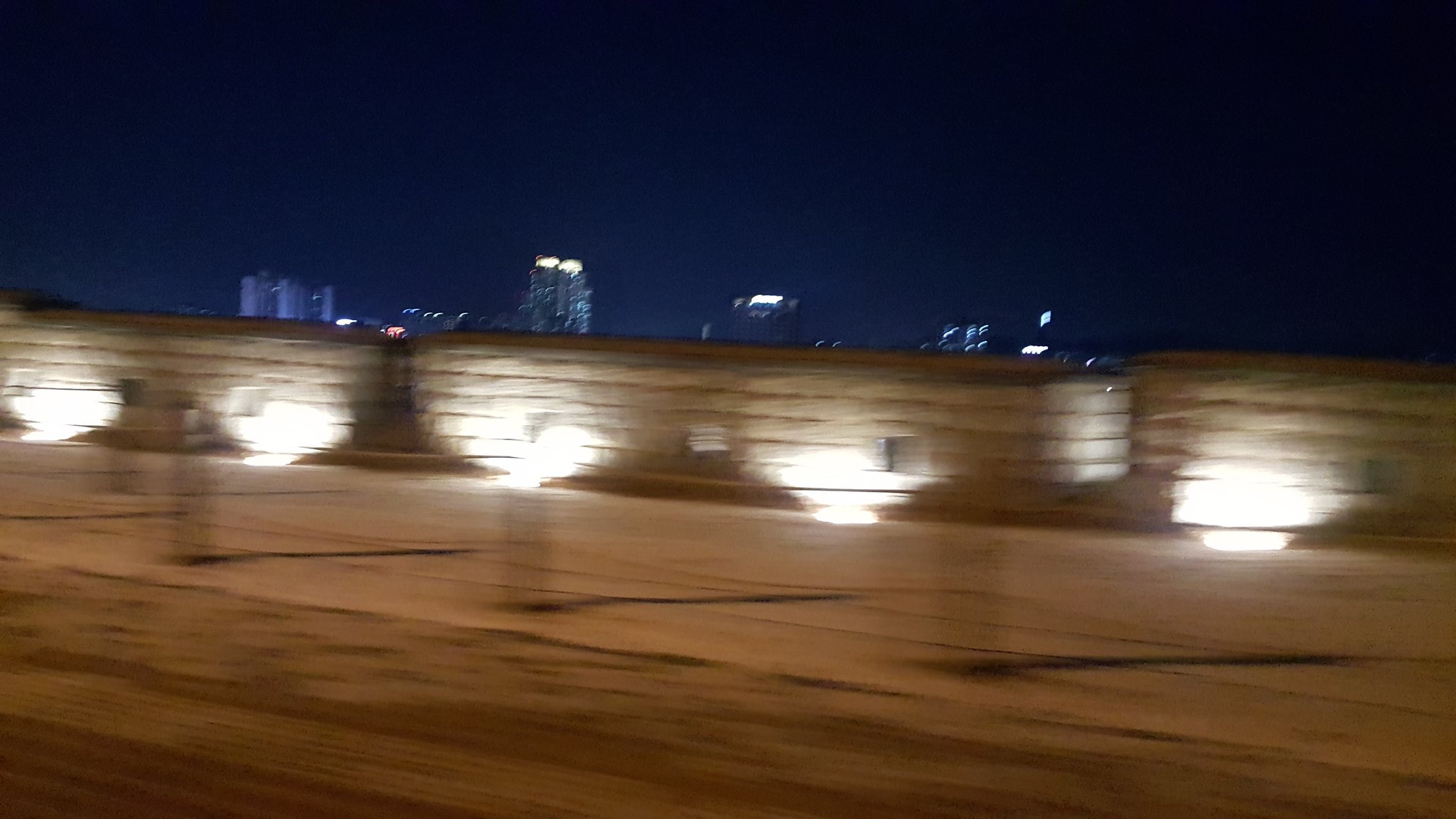The photo captures a night scene with a dark sky devoid of the moon or stars. A stacked, light gray brick wall with a tan top runs horizontally across the image, slightly angled upward towards the left. This wall is illuminated by five white lights evenly spaced along its base. Behind the wall, the tops of several skyscrapers with various white lights are visible, peeping over its edge against the darker blue and black gradient of the sky. The foreground is highly blurred, obscuring details but appearing to include a sidewalk and blurred black poles, with possible road elements closest to the camera. The overall image suffers from horizontal motion blur, making the background buildings more distinguishable than the indistinct objects in the foreground.